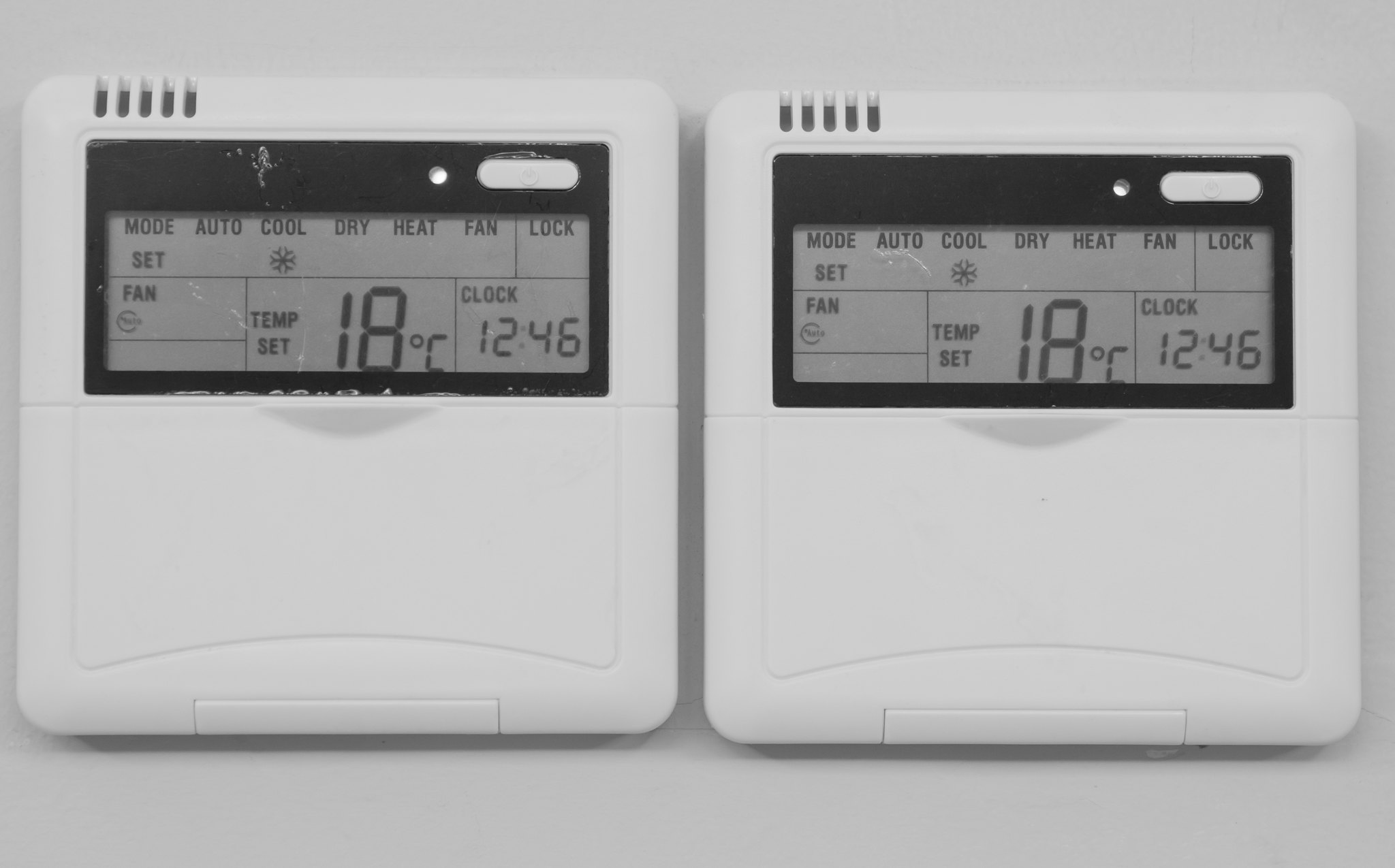This photograph features two identical air conditioning control units, designed to monitor and regulate temperature. Both units are sleek and white, and they are set against a white-gray background. 

Each control unit is square-shaped. On the top left corner of each unit, there are five small, rice-shaped holes that likely function as sensors. Below these sensors is a rectangular screen with a black border that occupies the top half of the square frame. 

The screen displays several indicators and settings: "Mode", "Auto", "Cool", "Dry", "Heat", "Fan", "Lock", and "Set". There is also a snowflake icon indicating the cooling mode. Beneath these indicators are additional readouts: "Fan", "Auto", "Temp Set", showing "18°C", and "Clock", displaying the time "12:46".

The bottom half of each control unit appears to be designed to flip open, evidenced by a small handle that can be pushed down. This suggests that there are likely more controls or settings hidden behind this panel.

The overall design is clean and functional, exhibiting a balance between aesthetic simplicity and technological efficiency.